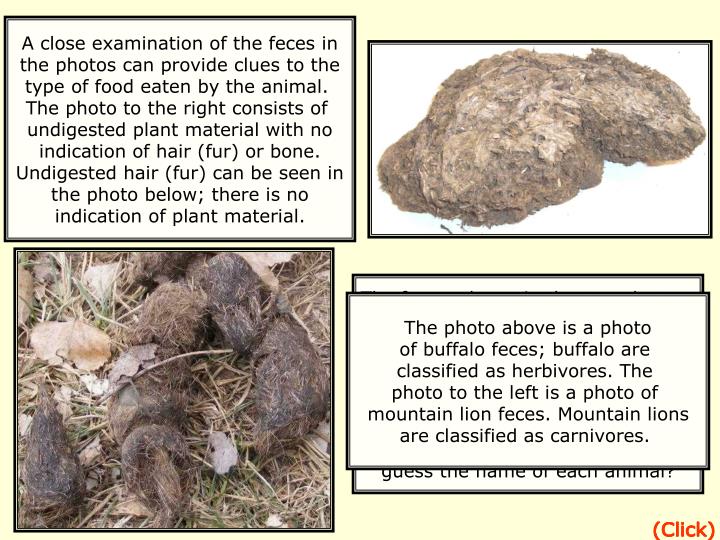This PowerPoint slide features a detailed comparison of buffalo and mountain lion feces, highlighting their dietary distinctions. The slide is divided into four black-outlined sections on a light yellow background. The top left section contains text explaining that analyzing feces can reveal dietary clues. The top right section displays a close-up of buffalo feces, which is brown with light spots and set against a white background. The bottom left section shows another sample of buffalo feces, this time on old grass with notable undigested hair, indicating herbivorous consumption. The bottom right section of the slide includes text identifying the photos: the top right image as buffalo feces—classified as herbivorous—and the bottom left image as mountain lion feces—classified as carnivorous. The slide also features a clickable red link in the bottom right corner.